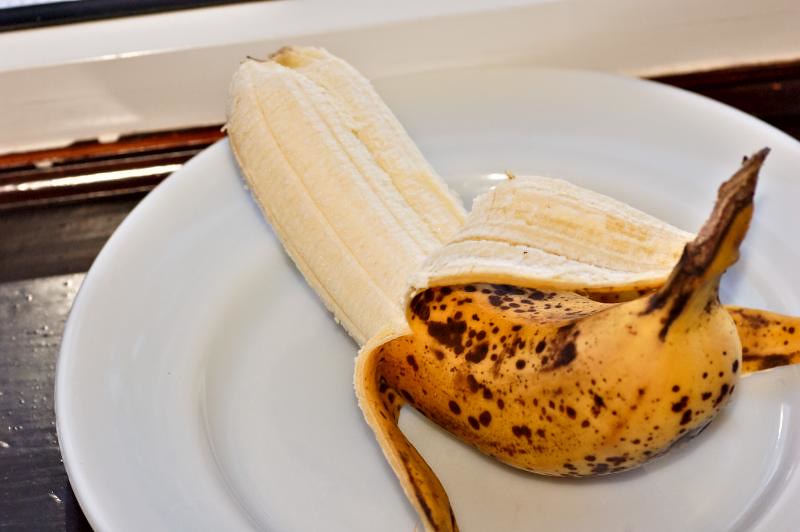This photograph captures a close-up view of a partially peeled banana resting on a white, circular plate. The banana, which appears slightly old with brown spots marring its yellow peel, lies on its side. The stem points towards the top right corner of the image, while the other end points towards the top left. The banana itself is unusual, giving the impression of two bananas fused together into one, which adds a unique twist to the otherwise simple subject. The plate is placed on a brown-painted surface, likely a windowsill, and the bottom of a white window frame is visible in the background. The overall setting suggests a casual, domestic environment, highlighting the oddity of the banana against a mundane backdrop.